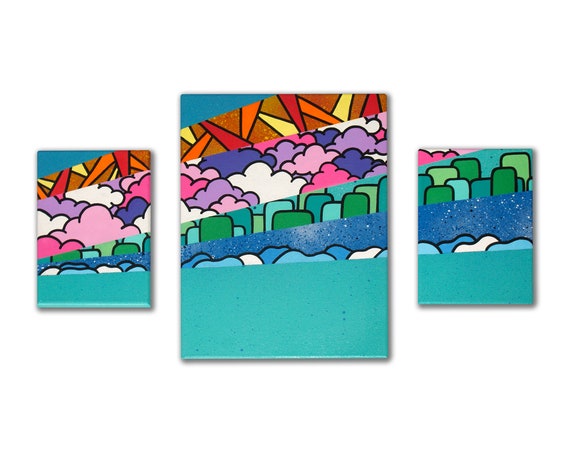This horizontal image features a series of three rectangular, colorful, abstract paintings, mounted against a white background. The central painting is the largest, flanked by two smaller, identically-sized paintings on either side. Each piece shares a similar composition: the lower portion is dominated by an aqua blue color, transitioning into various abstract shapes and hues above.

In the central painting, an aqua-colored foreground gives way to what appears to be an abstracted train, with blue bottom sections resembling train cars and green protrusions possibly representing trees or buildings. Above this, the "sky" is a vibrant mix of clouds in pink, blue, white, and purple hues. The topmost section contains an array of abstract shapes, adding depth and complexity to the composition.

The side paintings mirror the central one but in reduced and slightly varied forms. The left painting maintains the same color scheme and elements but in a condensed version, while the right painting focuses more closely on the abstract forms at the base, dominated by the same aqua blue and green elements, without extending to the full sky and top section found in the center.

Overall, the trio forms a cohesive, dynamic display of abstract art, rich in colors like aqua, blue, green, pink, purple, and white, with the central piece offering a more expansive view, and the side paintings providing complementary close-ups.